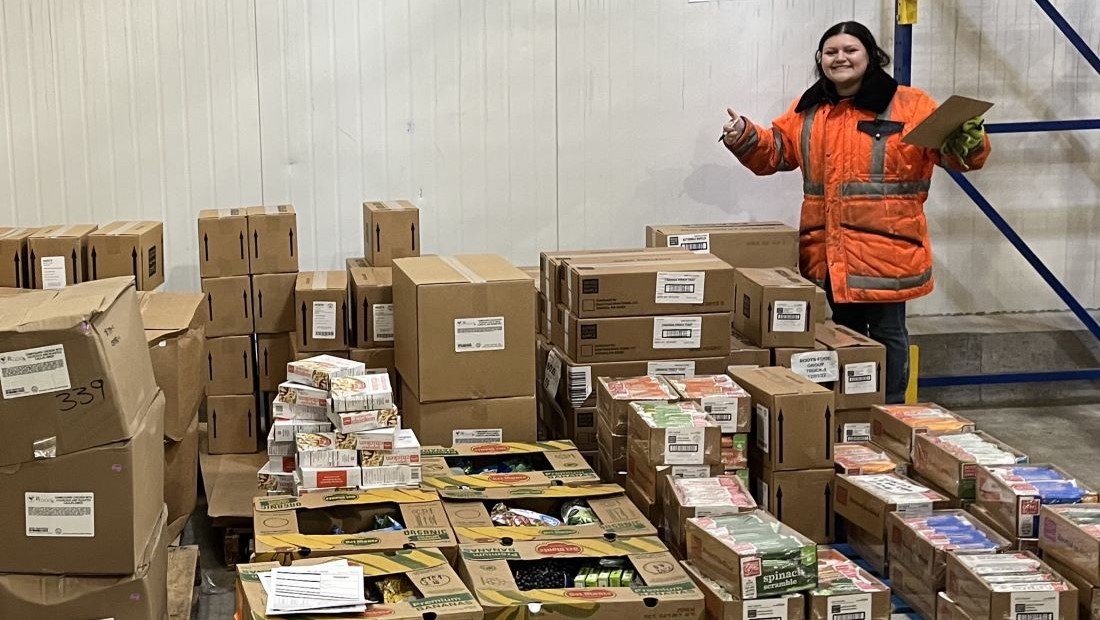In this photograph taken inside a warehouse, we observe a bustling scene centered around a multitude of cardboard boxes, many of which are open and revealing their contents. The boxes, primarily brown with some featuring spinach and other non-perishable foods, span from the left side of the image to nearly the right. Some have labels with barcodes and appear to be standard banana and white boxes used for storage and logistics. In the upper right, a young woman stands beside the boxes. She is sporting a heavy, orange, high-visibility jacket with grey reflective stripes and a thick black collar. Her outfit is completed with yellow gloves. She holds a pen in her right hand and a brown clipboard in her left, while giving a thumbs up and smiling. The setting appears to be a food drive or a food bank operation, with white metal walls and concrete floors framing the background of this industrious scene.